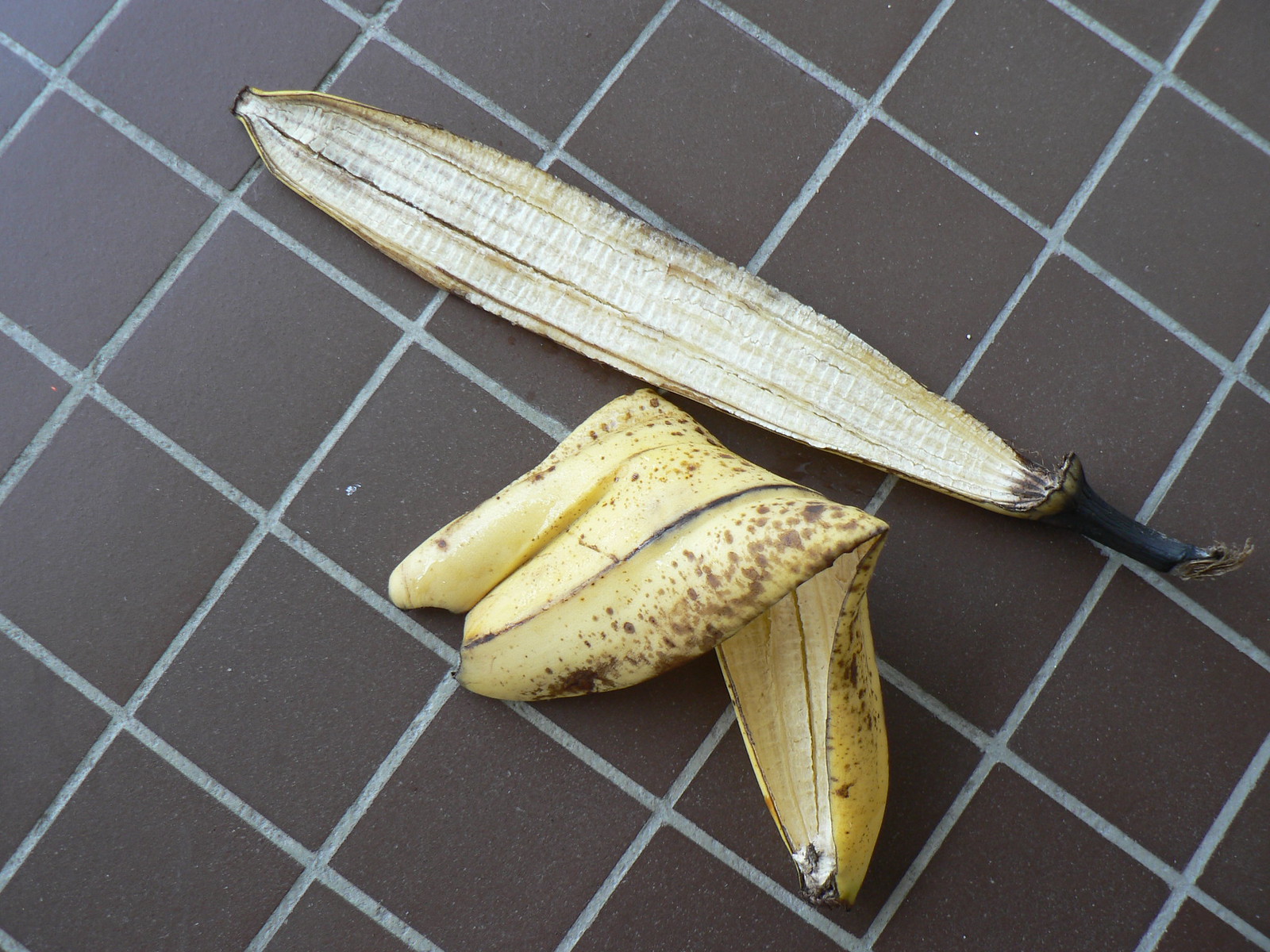A single banana peel is meticulously laid out on a brown ceramic tile surface, each tile square-shaped with gray grout lines. The primary section of the peel, complete with its stem, is positioned diagonally from the upper left to the lower right corner. This portion, showing the inner side of the peel that once hugged the banana, spans approximately four tiles in length. Below it lies the remaining portion of the peel, appearing as if the banana was peeled in three additional sections yet still attached at the base. This part of the peel is bent backward, exposing its outer yellow skin side down at first, then curving back to reveal the vibrant yellow on top. This final bend directs diagonally towards the lower left-hand side of the image, creating a visually striking composition against the tiled background.